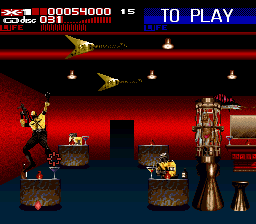The image depicts a scene from a video game featuring a character standing on a platform located on the left side of the frame. The game environment includes a total of four platforms: two in the foreground and two in the background. Suspended in the air above these platforms are several flying, gold-colored items. The ceiling of the room is adorned with four lights, beneath which a score of 54,000 is displayed prominently at the top left corner of the image. Adjacent to this score, towards the right, the number 15 is visible. Further right, there is white text against a blue background that reads "To Play," accompanied by a small blue rectangular label.

The room itself reveals two visible red walls, and in the distant background, an open doorway can be seen on the back wall.